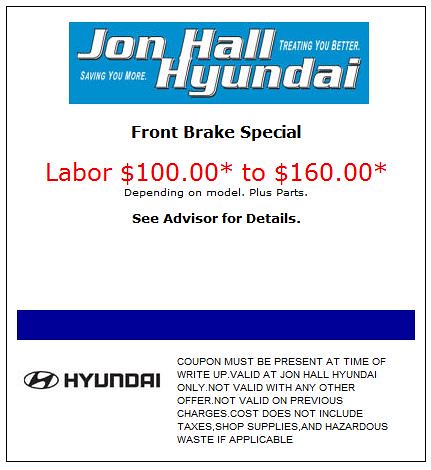The image features an advertisement for John Hull Hyundai, predominantly set on a white background. At the top, there is a blue rectangular box containing the text: "John Hull Hyundai, treating you better, saving you more". Just below this box, the text reads: "Front brake special, labor $100.00 to $160.00 depending on model plus parts". Further down, there is a dark blue horizontal strip beneath which, on the left side, sits the Hyundai logo. On the right side of this strip, detailed disclaimers are provided: "Coupon must be present at time of write-up. Valid at John Hull Hyundai only. Not valid with any other offer. Not valid on previous charges. Cost does not include taxes, shop supplies, and hazardous waste if applicable."